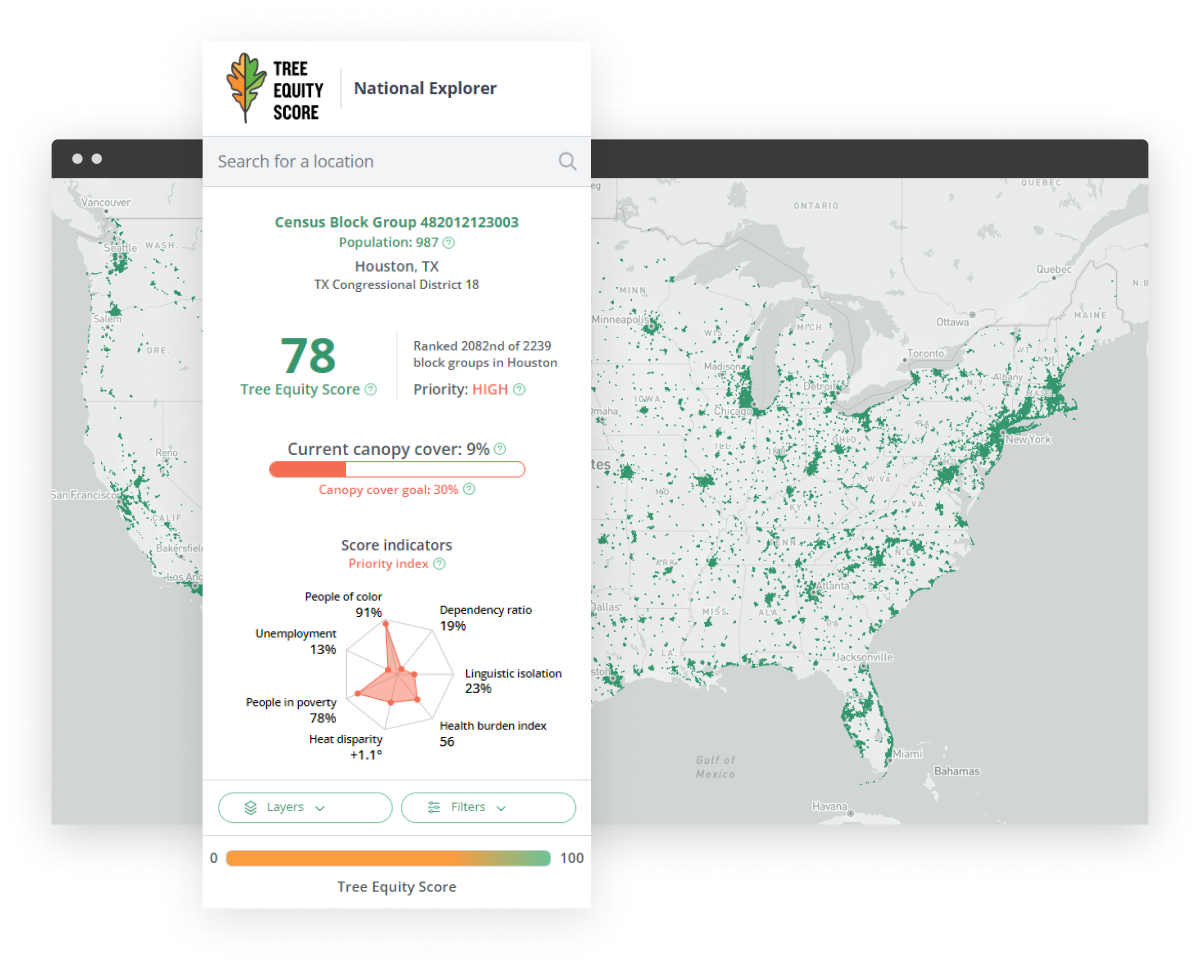The image depicts a detailed map of the United States with a predominantly gray background. Scattered across the map, various areas are highlighted in green. Overlaying the map, there is an interface element featuring a gray search box at the top with the prompt, “Search for a location.” Beneath this, text reads, “Census Block Group 48 201 21 23 0 0 3 Population,” though the full contents are partially obscured and not fully legible.

In the upper section of the overlay, the image indicates “Houston, Texas, Congressional District 78,” accompanied by a tree equity score with a priority level marked as "High." The current canopy cover is noted to be 9%, with a goal of increasing to 30%. Additional details include various score indicators. At the bottom of the interface element, there are tabs labeled "Layer" and "Filters." The overall layout suggests a focus on environmental metrics and urban planning insights for a specific geographic region.